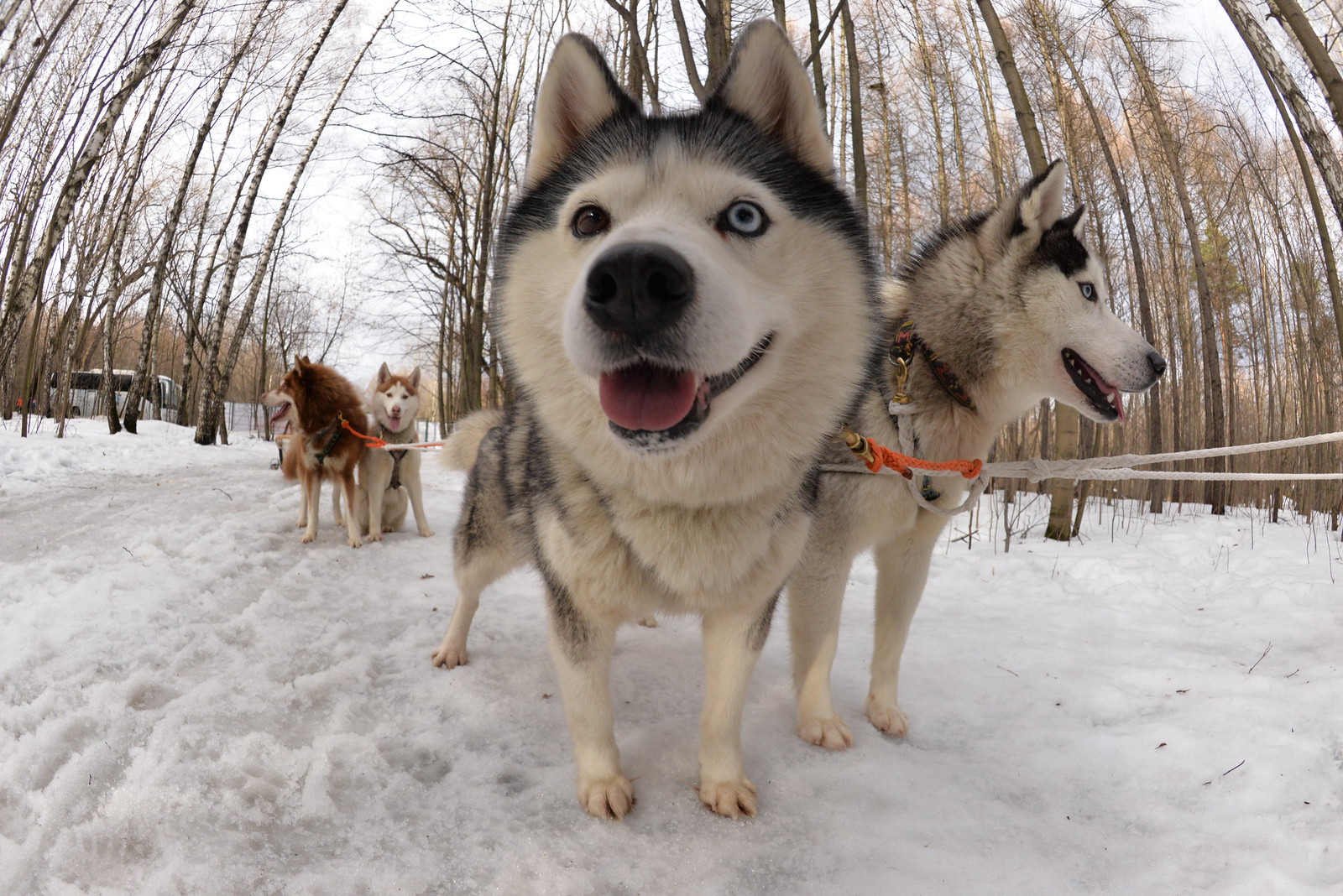In a picturesque, snowy scene, a team of four huskies stands alert and ready. Two pairs of dogs line up, with the front pair prominently featured. Each of these front-row huskies has striking blue eyes, one with mismatched eyes—one a captivating blue and the other a warm brown. The second dog in the front turns its head, showing off its singular blue eye. Coats of white combined with darker shades adorn these front two huskies, contrasting with the warm brown fur of the pair behind them. They are tethered together with white ropes, hinting at the presence of a sled just out of the frame. The snowy ground is littered with footprints, suggesting recent dog traffic. Barren trees form a natural canopy, creating a tunnel-like formation in the background. To the far left, a white vehicle is parked, adding a modern touch to this wintry landscape. The dogs, looking content and alert, are surrounded by the pristine beauty of a winter day.